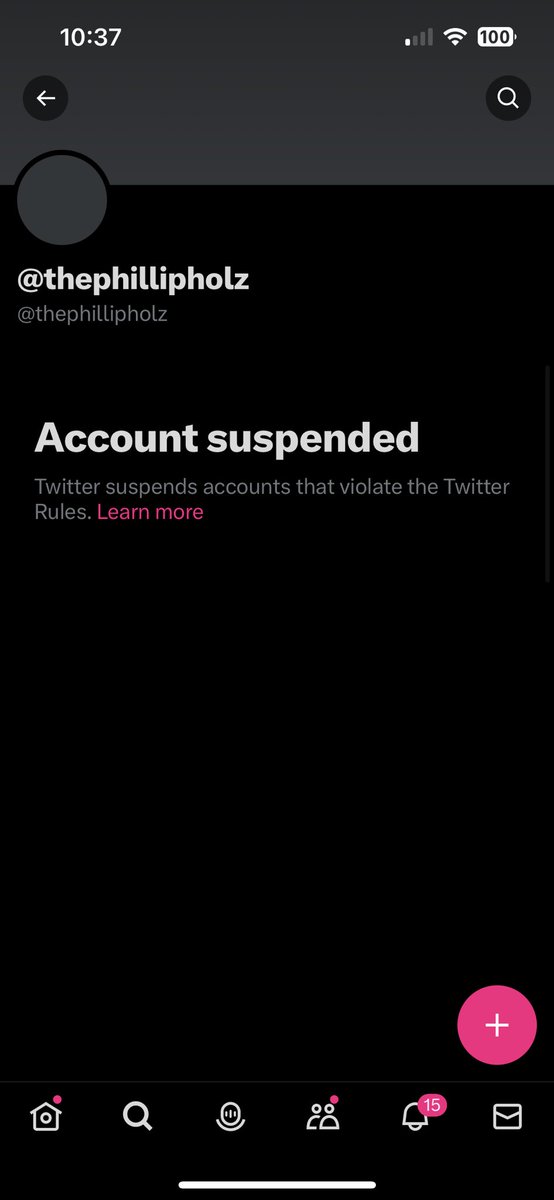This image captured on someone's phone demonstrates a suspended Twitter account interface. At the top of the screen, the battery is fully charged at 100%, displayed in the upper right-hand corner, while the time reads 10:37 in the upper left-hand corner. The predominant color of the background is black, indicating a dark mode display. The top banner is dark gray, maintaining the somber tone of the alert. The username visible is "ThePhilipHoles," accompanied by the handle @ThePhilipHoles, with a profile picture represented by a plain dark gray circle.

Central to the image is the bold message "Account Suspended," indicating that the account has been flagged for violating Twitter's rules. Beneath this title, a smaller text explains, "Twitter suspends accounts that violate the Twitter Rules." A pink "Learn More" link provides additional information regarding the suspension. At the bottom of the screen, standard Twitter navigation icons are visible, including the homepage, search bar, microphone, friends, notifications, and email. Additionally, a pink plus sign in the lower right-hand corner suggests the option to compose a new tweet or post.